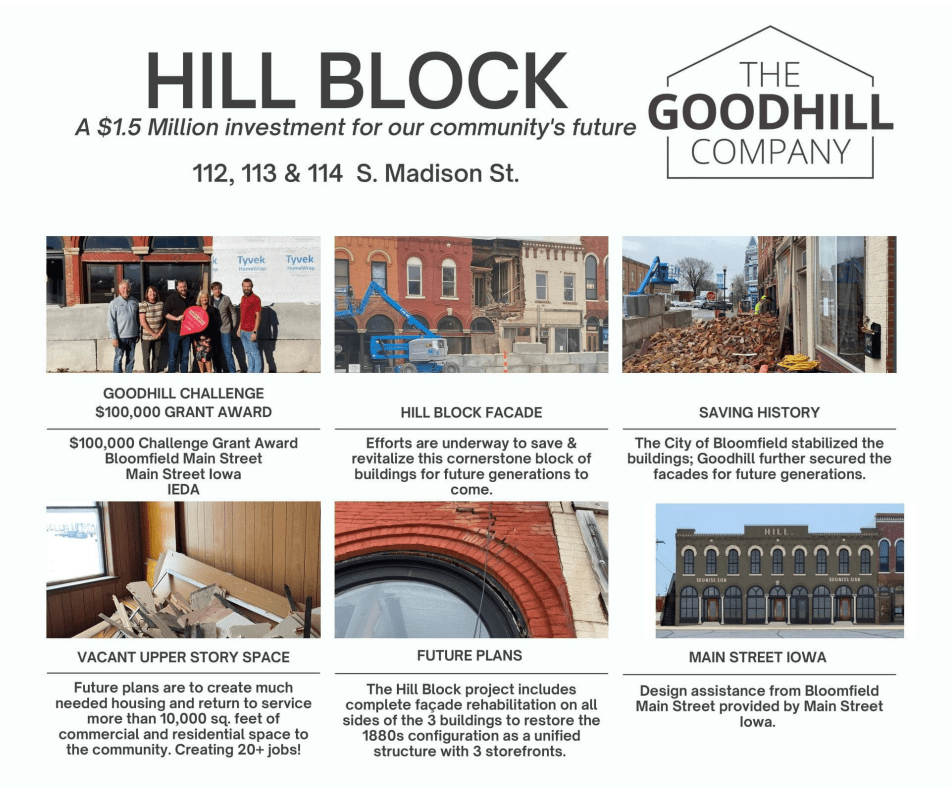The image is an advertisement from the Good Hill Company, featuring their $1.5 million investment titled "Hill Block: A $1.5 Million Investment for Our Community's Future." The project focuses on the revitalization of three addresses on South Madison Street, specifically 112, 113, and 114. The advertisement includes six images depicting the renovation efforts and progress, both of the people involved and the buildings themselves. One highlighted initiative is the Good Hill Challenge, which awarded a $100,000 grant to Bloomfield Main Street in Iowa. The narrative of the Hill Block Project emphasizes the importance of saving historical buildings, securing their facades, and rehabilitating them for future use. The initiative includes plans to convert vacant upper-story spaces into much-needed housing and commercial areas, aiming to add over 10,000 square feet of usable space and create more than 20 jobs. The design assistance for this project is provided by Bloomfield Main Street in collaboration with Main Street Iowa.